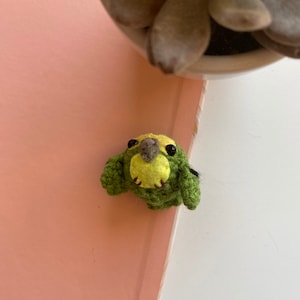This photograph showcases a small toy resembling a bird, crafted predominantly from green crocheted yarn. The bird features a brown beak and two black bead-like eyes. Its head is adorned with yellow felt, both on the top and bottom, contributing to its charming, lifelike appearance. The toy rests on a split-colored surface, pink on the left and white on the right, adding a visually appealing backdrop. Above the toy bird, in the upper right corner of the image, sits a decorative clay or wooden pot containing a brown succulent plant. The scene is captured from a top-down perspective, with the crocheted bird toy being the central focus.